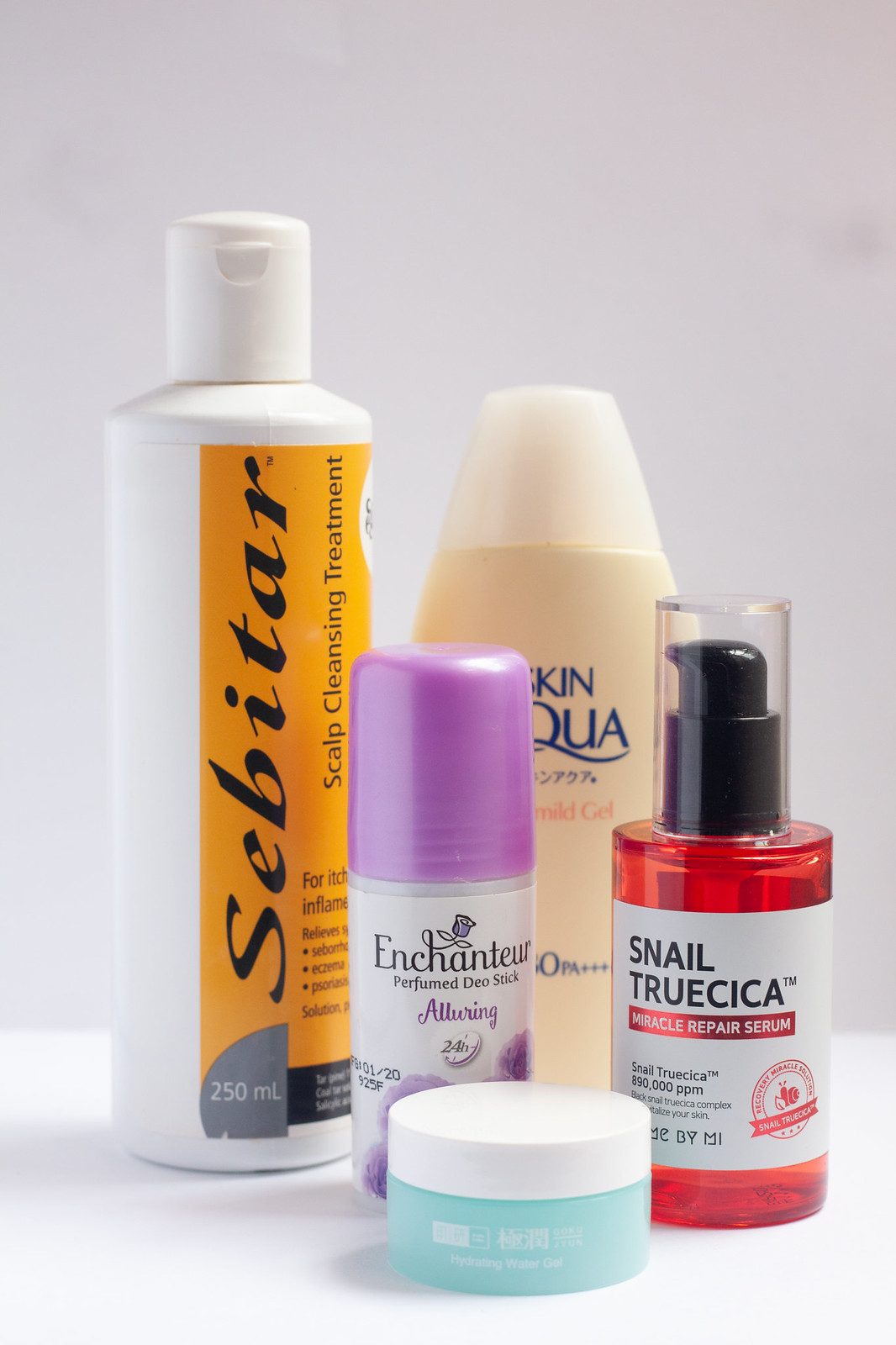The image displays an array of five different cosmetic products arranged on a pristine white table, set against a clean white background. 

From left to right:

1. The first product is a tall, slender white bottle with a matching white lid, prominently featuring an orange label with black text. The label reads "SEBITAR Scalp Cleansing Treatment for Itch, Inflammatory Relief, Eczema and Psoriasis Solution." It also indicates a volume of 250 milliliters in a gray section with white text.

2. Positioned next to it is a significantly shorter, white aerosol can adorned with black and purple text and capped with a purple lid. This product is labeled "Enchanture Perfumed Deo Stick Alluring 24 Hours," and is decorated with an illustration of purple flowers, although the specific scent isn't identifiable.

3. In the front center of the image is the smallest item: a squat, shallow container resembling a holder for pimple pads. It features a frosted blue base with a white lid. The label on this item reads "Hydrating Water Gel."

4. To its right stands a sleek, translucent red bottle equipped with a black pump dispenser. This item boasts a white label with black text, describing it as "Snail True Cica Miracle Repair Serum" and highlighting its content with "Snail True Cica, 890 ppm" and "Black Snail True Cica Complex for Vitalize Your Skin and Recovery."

5. The final product, situated in the very back, is a wider bottle that appears to be a shampoo bottle. It’s partially obscured, but it seemingly bears the name "Redken Aqua." This bottle is pale cream in color and features writing in blue and orange, with the orange text indicating it is a "Mild Gel."

Overall, this image showcases a curated selection of skincare and personal hygiene products, giving insight into the user's daily cosmetic routine.